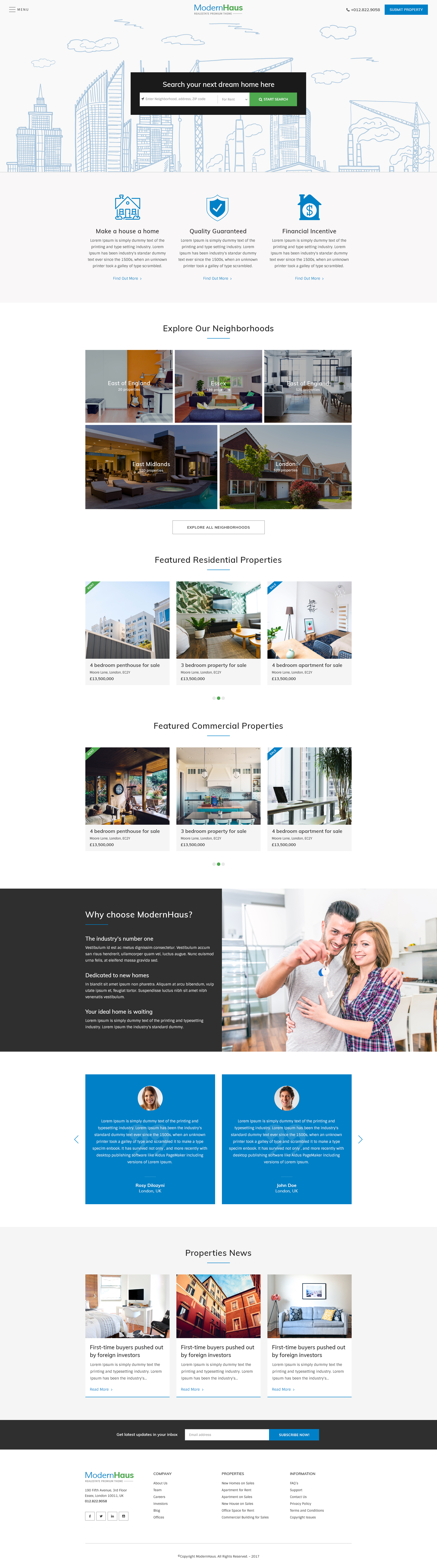The image depicts an interface for purchasing or building a home. At the top, it prominently features the title "Modern House HAUS" in green text, accompanied by a hand-drawn illustration of a city skyline, including a skyscraper. Below this, there's a search box and several icons with labels such as "Make a House a Home," "Quality Guaranteed," and "Financial Incentive."

Further down, the interface invites users to "Explore a Neighborhood," displaying five pictures of various residential areas. It then highlights sections for "Featured Residential Properties" and "Featured Commercial Properties." Another section titled "Why Choose Modern House?" includes an image of a man and woman holding a set of keys, suggesting they have just purchased a home. These same individuals appear again in a feedback section, though the text is too densely packed to read clearly.

The "Property News" section features three images: one of a couch against a tan wall (on the right), an apartment building (in the middle), and a computer in a living room setting (on the left). Additional menu options are listed below these, culminating in a black box containing a button labeled "Subscribe."